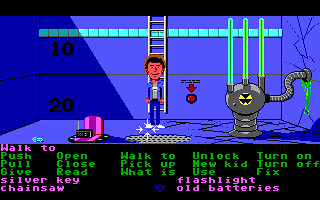This image captures a scene from a retro-style video game, likely from the late 1980s or 1990s, laid out in a horizontal or landscape orientation. The central focus is a character dressed in a blue jacket, dark blue trousers, a white t-shirt, and white shoes, standing on a blue floor. He is positioned in front of a gray ladder against a matching blue wall with numerical markings "10" and "20" on the left side. On the bottom left corner is a pink item, potentially a laptop, with black text on it.

On the right side of the character, a gray machine with a yellow and black warning sign and three vertical green rods is visible. This machine connects to the wall via a flexible pipe leaking green liquid. Additionally, there is a prominent red button with a red arrow pointing towards it.

The bottom of the screen features a black panel with various commands and interactions in green and pink text. On the left, it lists options such as "Walk To," "Push," "Pull," "Give," "Open," "Close," and "Read." Beneath these commands are labels like "Silver Key" and "Chainsaw." Centering the bottom panel, green text indicates "Walk To" and "Pick Up." To the right, the options "Unlock," "New Kid," "Use," "Turn On," "Turn Off," and "Fix" are displayed in green, with "Flashlight" and "All the Batteries" in pink below them. A blue downward-pointing arrow is located at the bottom center.